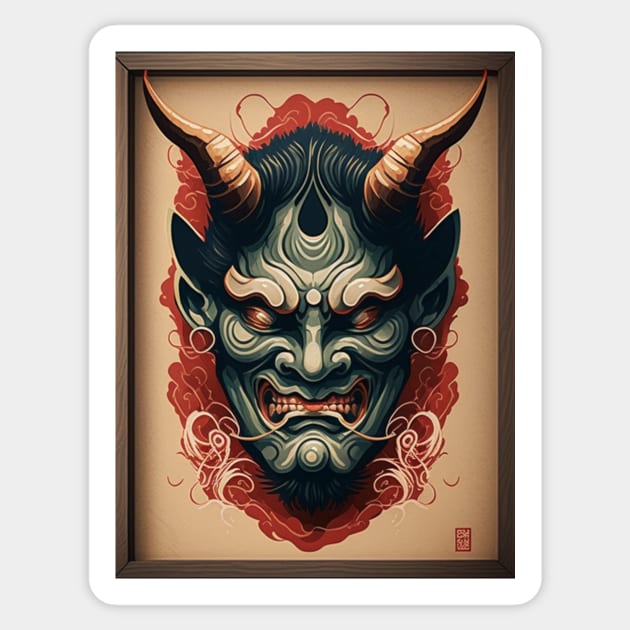This framed image depicts a striking, stylized representation of a devil that appears both frightful and captivating. The frame consists of a thin wooden border surrounding a gray rectangle, slightly taller than it is wide, with a white inner border, hinting that this could be a photograph of artwork. Set against a beige or khaki background, the image centers on a devilish face reminiscent of a Japanese kabuki theater demon mask.

The devil has a deep green or grayish-teal complexion, adorned with intricate white swirls and tattoos. Piercing red eyes feature black stripes, and its mouth, filled with a full set of white teeth, is accented by red, giving an impression of blood. Two horns protrude from the top of its forehead, transitioning in color from black at the base to brown at the tips. The devil's ears are pointed and elf-like, starting black near the eyes and fading to gray.

The face is framed by an aura of red, cloud-like swirls, and black hair surrounds the head and chin, adding to its menacing appearance. White furry eyebrows and whisker-like white curls emerge amidst the vibrant red aura. The lower right-hand corner of the image contains what seems to be a block print attribute, possibly a red square with characters, suggesting some cultural or artistic significance to the artwork's origin. The overall depiction is far from pleasing but holds an intriguing allure for those drawn to such vivid and dramatic representations.